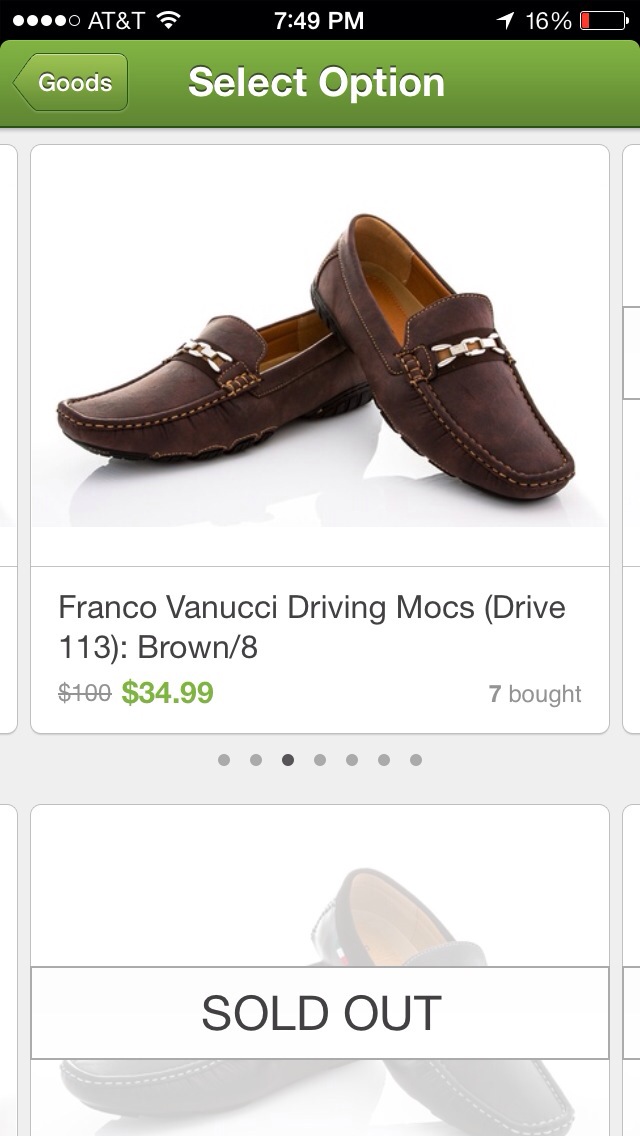The image appears to be a vertically aligned screenshot taken from an iOS device at 7:49 PM with an AT&T network and 16% battery remaining. The interface shows a webpage with a green banner reading "select option" and a back arrow button to the left. Below the banner, a centered white background displays a pair of brown moccasin-style loafers with gold buckles and detailed front stitching, angled slightly atop each other. These shoes are labeled "Franco Vannucci Driving Mocs (Drive 113), Brown/8" with a price tag of $34.99, marked down from $100. Additionally, the notation "7 bought" is displayed. Underneath this, a faded duplicate image of the same shoes appears with a "sold out" label across it. The colors in the image include shades of brown, gold, green, and elements of red, white, black, tan, grey, and silver.